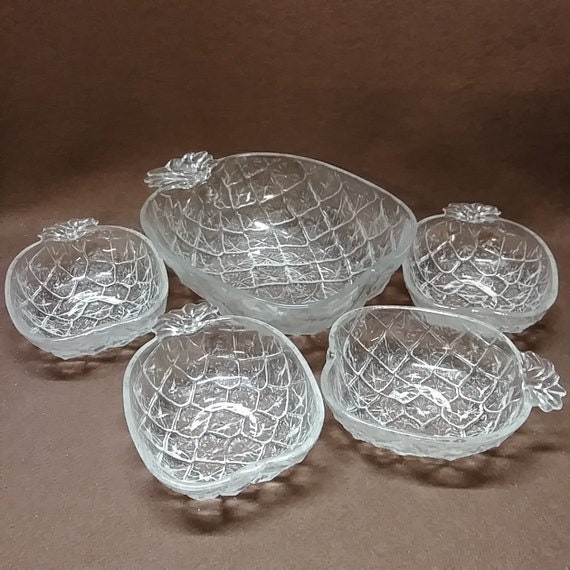This professionally taken, square photograph features a set of five clear glass pineapple-shaped serving dishes arranged on a dark brown surface, set against a grayish-brown, indistinct background. The set consists of one larger serving dish in the center and four smaller bowls surrounding it. Each piece of glasswork mimics the texture and form of a pineapple, including a leafy stem and a patterned exterior resembling pineapple skin. The transparent glass is slightly reflective, casting distinct shadows beneath each dish where the textured patterns are visually echoed on the surface below. These decorative and functional glass bowls are likely intended for serving fancy meals or holding items like candy on a coffee table, and the photograph appears to be used for advertising or selling the set.